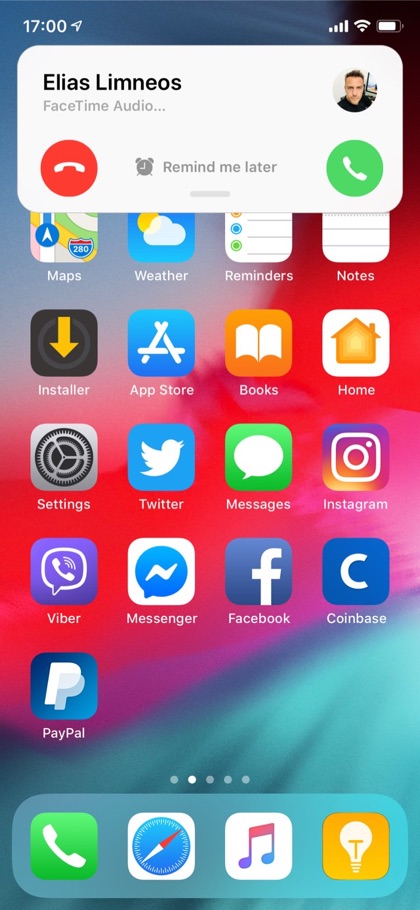In this screenshot of a cell phone, the background showcases a gradient that transitions from a light blue at the bottom, to pink and red in the middle, and finally to a dark blue at the top, resembling the colors of the sky. 

At the top left corner, the time is displayed as 17:00 hours, alongside an arrow. The top right corner shows full cell signal strength, full Wi-Fi signal, and an almost full battery icon.

Below, an open tab is visible with a white background and black text that says "Elias Lemonade" with an image of Elias on the far right. Beneath "Elias Lemonade," the text reads "FaceTime Audio." 

Towards the bottom, there are three buttons: a red background button with a white phone icon, labeled for ending a call; a "Remind Me Later" button with an alarm clock icon in the middle; and a green background button with a white phone icon for accepting a call.

Further down, various app icons are arranged in several rows including Maps, Weather, Reminders, Notes, Installer, App Store, Books, Home, Settings, Twitter, Messages, Instagram, Viber, Messenger, Facebook, Coinbase, and PayPal.

At the very bottom, docked icons include a green Phone icon, a Compass icon, a Music icon, and a yellow box with a white light bulb and the letter T, both in yellow.